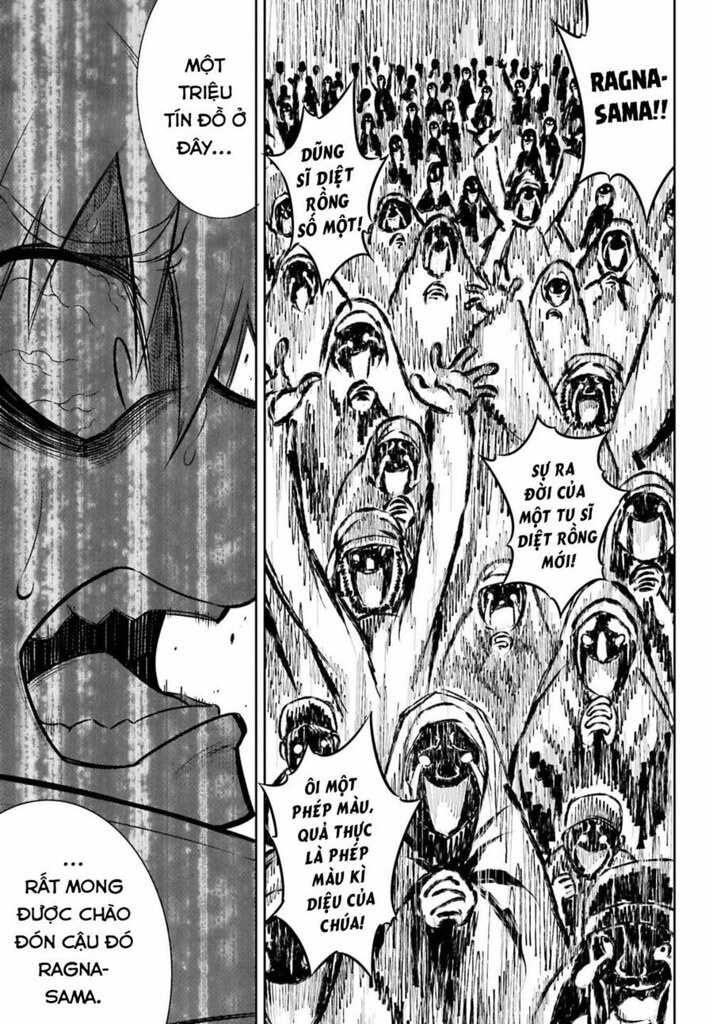The image appears to be taken from an Asian comic book or anime, featuring a layout split into two main panels. The left panel, occupying about a quarter of the page, provides an intense close-up of an anime-style character who appears to be in a state of anxiety or fear, with features such as a bulging eye partially obscured by hair, a sweat-drenched face, and an open mouth suggesting they've just seen something alarming. The larger right panel, covering approximately 75% of the page, depicts a crowd of people who are energetically raising their hands in the air, possibly cheering, laughing, or crying, with expressions that indicate a high level of excitement or distress. They are all exclaiming something that is unreadable due to the language barrier. The crowd includes individuals that might be interpreted as wearing white gowns and masks, giving them a somewhat ominous presence.